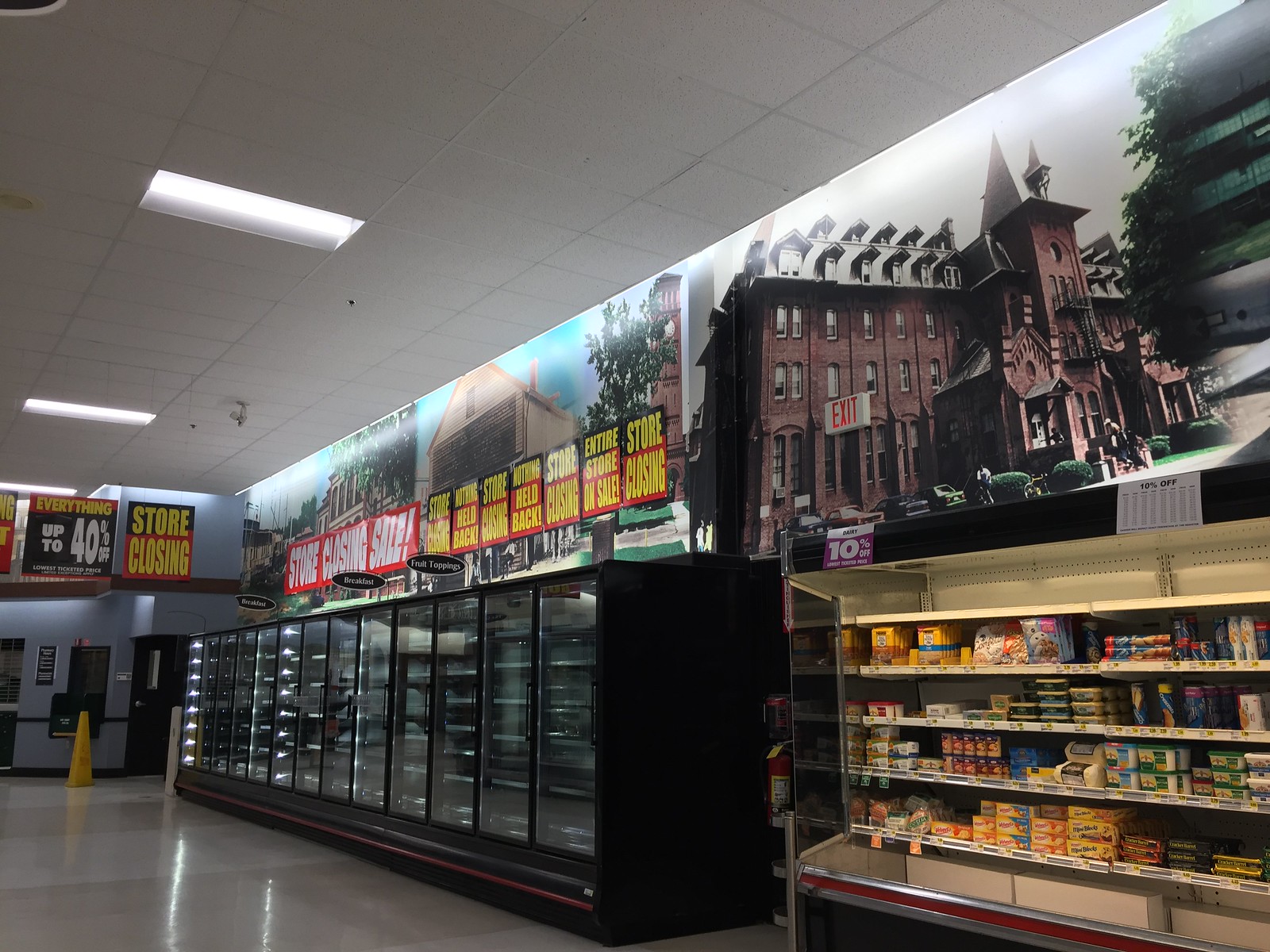This image depicts a section of a supermarket that is in a state of closure. The store features a gleaming floor that reflects the overhead illumination coming from large, white, window-like lights embedded in the tiled ceiling. On the right side, there is a freezer section stocked with various cheeses, butter, and pre-made baking products, such as frozen cookie dough ready to be baked. Adjacent to this are about ten rows of freezer drawers, which appear notably sparse and nearly empty.

Throughout the area, prominent signs announce the imminent closure of the store, proclaiming that everything is up to 40 percent off as part of a store-wide sale. The left side of the image captures more freezer units, mostly devoid of goods, reinforcing the impression of an extensive inventory clearance. The overall scene conveys a sense of finality and transition, as this supermarket prepares to shutter its doors for good.